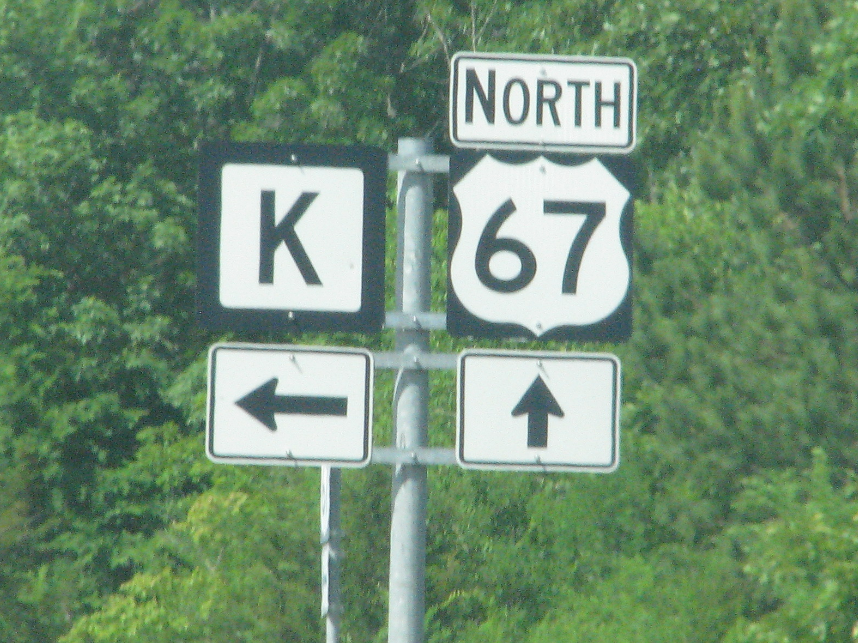The image appears to be taken from a moving car, capturing a close-up view of highway signage. Central to the photo is a metal post adorned with several street signs. On the top-left is a sign with the letter "K," and directly below it is a sign featuring a left-pointing arrow. To the top-right, there's a shield-shaped sign emblazoned with the number "67," indicating a highway route. Below the shield, a sign with an upward-pointing arrow can be seen. Above the "67" highway sign, an additional label indicates the direction "North." The background is lush with green trees, filling the frame and hinting at a roadside scenery.